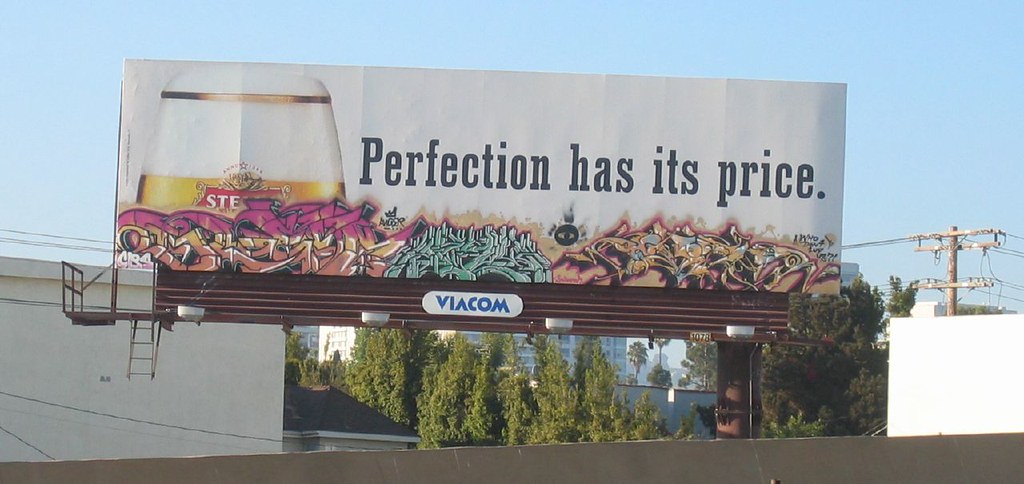This image portrays a distant view of a billboard set against a vibrant, clear blue sky. To the right of the billboard, an old telephone pole is visibly detailed, featuring two sections from which the lines extend. The billboard itself has a white background. On the left side of the billboard, there is an image of a clear glass adorned with a golden rim. The glass is filled with an amber-colored liquid, featuring the letters "S-T-A" in white, outlined in red. Bold black text across the billboard reads, "Perfection has its price." Below this text, various colors are artistically strewn, including shades of gold, pink, green, combined with brown and a hint of blue.